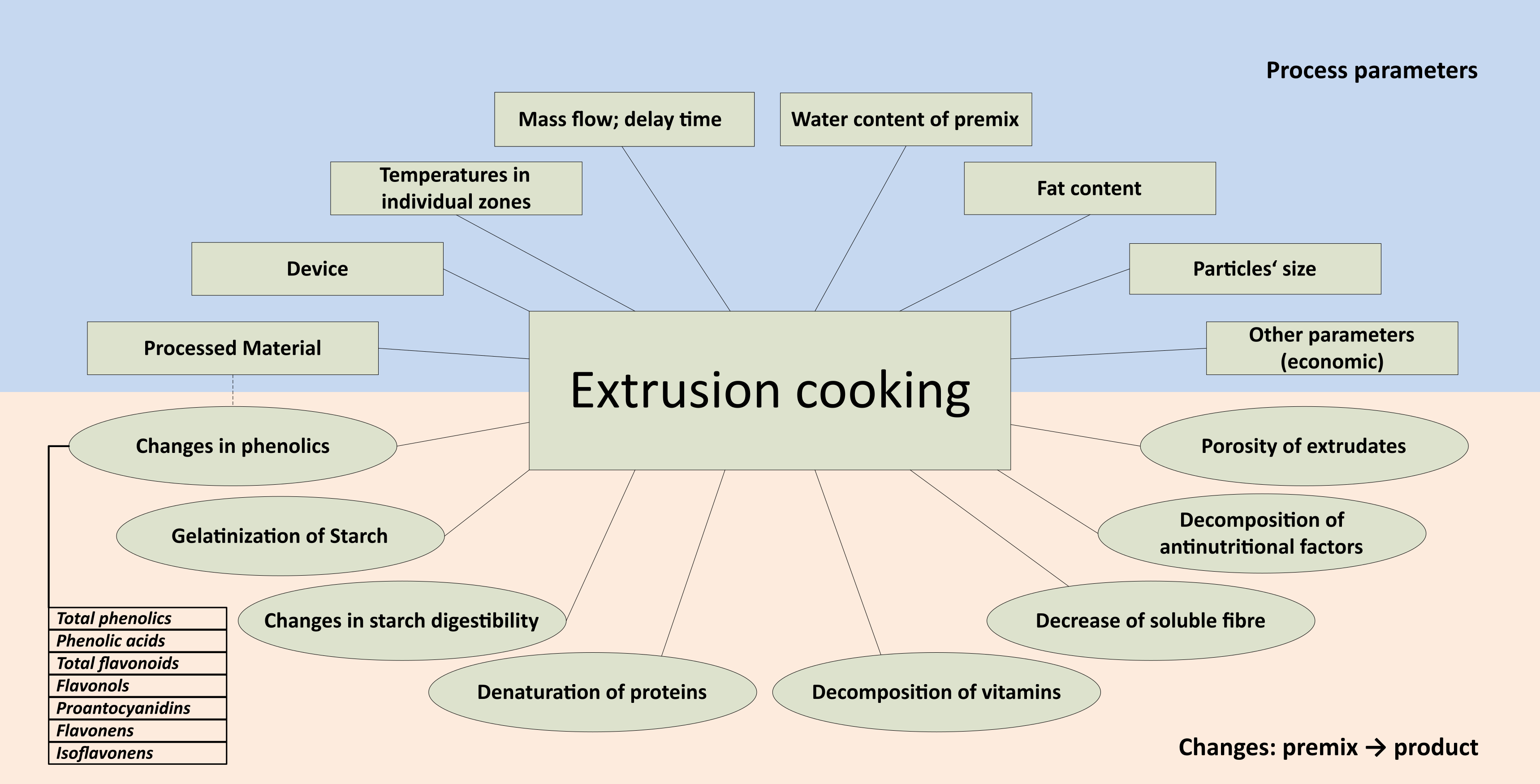The image appears to be a detailed process flow diagram titled "Extrusion Cooking," likely extracted from a book or similar reference material. In the center of the diagram, a green rectangular box, labeled "extrusion cooking" in black text, is prominently displayed. This central box is connected via arrows to several other rectangular and oval-shaped boxes, each illustrating various parameters and outcomes of the extrusion cooking process.

At the top half of the image, set against a blue background, seven rectangular bars list the process parameters: device, temperature in individual zones, mass flow delay time, water content of premix, fat content, particle size, and other parameters. The top right corner of this section highlights "process parameters" in black text. 

Moving to the bottom half of the image, which features a pale red background, a number of oval bubbles are linked to the central extrusion cooking box. These bubbles detail the changes and effects in the product, including the porosity of extrudents, decomposition of anti-nutritional factors, decrease of soluble fiber, decomposition of vitamins, denaturation of proteins, changes in starch digestibility, and gelatinization of starch. Moreover, another list in the lower left corner addresses additional components such as phenols.

Additionally, an arrow from an oval bubble on the bottom right indicates a transition labeled "changes premixed to product," summarizing the flow from the input materials to the final product. This comprehensive diagram visually maps out the intricate relationships between process parameters and the resulting transformations during the extrusion cooking process.